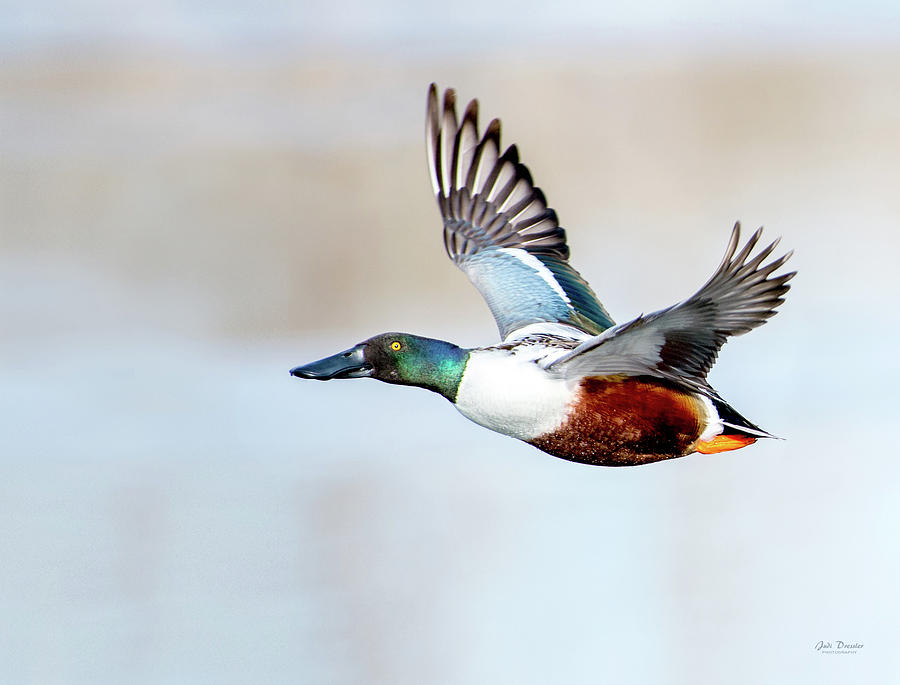This is a professional photograph capturing a northern shoveler or mallard duck in mid-flight against an artistically blurred background that transitions from blue at the bottom to brown at the top, suggesting a marsh or lake. The duck, perfectly in focus at the center, is displayed in exquisite detail. Its iridescent green head glows with a striking yellow eye and a broad black bill. The duck's neck and upper chest are white, transitioning to a rich orangey-brown band encircling its belly. Its wings, extended as it flies leftward, exhibit an intricate palette with black, white, blue, and green hues. Near the tail area, white and dark feathers blend seamlessly, while the orange webbed feet are tucked underneath. An out-of-focus artist's watermark and signature, unreadable due to its size, is visible in the bottom-right corner of the image, adding a professional touch to this stunning avian portrait.